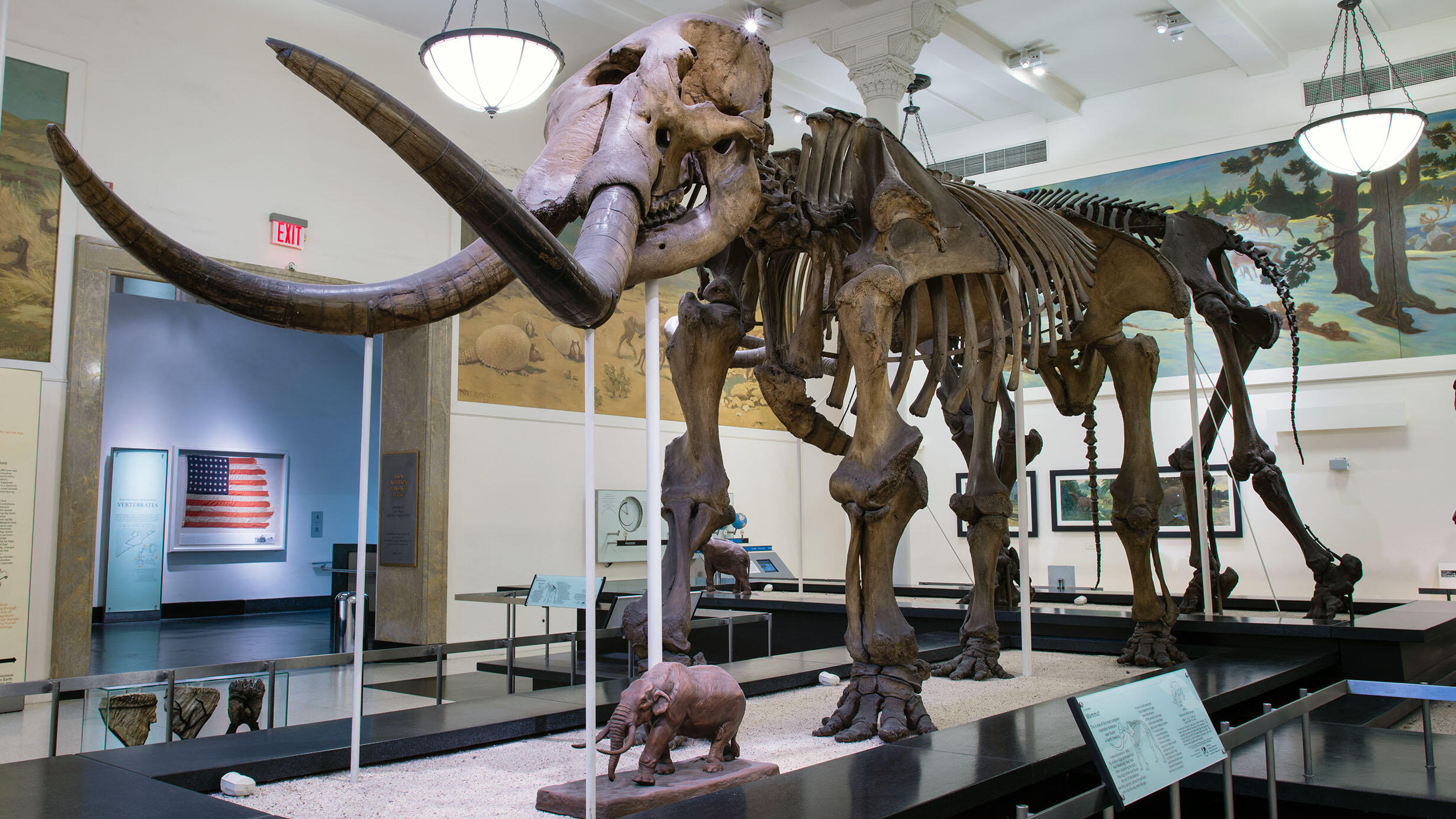The photo depicts a meticulously assembled exhibit in a museum, likely an educational institution, showcasing the skeleton of a large prehistoric mammal, possibly a mammoth, given the enormous, brown-grayish-yellow tusks extending from its skull. This significant centerpiece, supported by white rods, is fully reconstructed, emphasizing the impressive size and structure of the creature, which dwarfs the smaller ceramic statue placed beneath it to show what the animal might have looked like in life, albeit at a much smaller scale. The display appears to have been captured professionally, with excellent lighting highlighting the skeletal details and ensuring clarity of the surrounding environment. The backdrop features white walls adorned with various paintings and illustrations of geographical elements, a noticeable framed American flag, and hanging light fixtures from the ceiling, adding to the exhibition's educational ambiance. Additionally, a white sign laden with information about the mammoth is positioned near the skeleton, although its text remains indistinguishable in the photograph. The setting is devoid of people, allowing the focus to remain solely on the impressive skeletal display and the contextual elements that surround it.